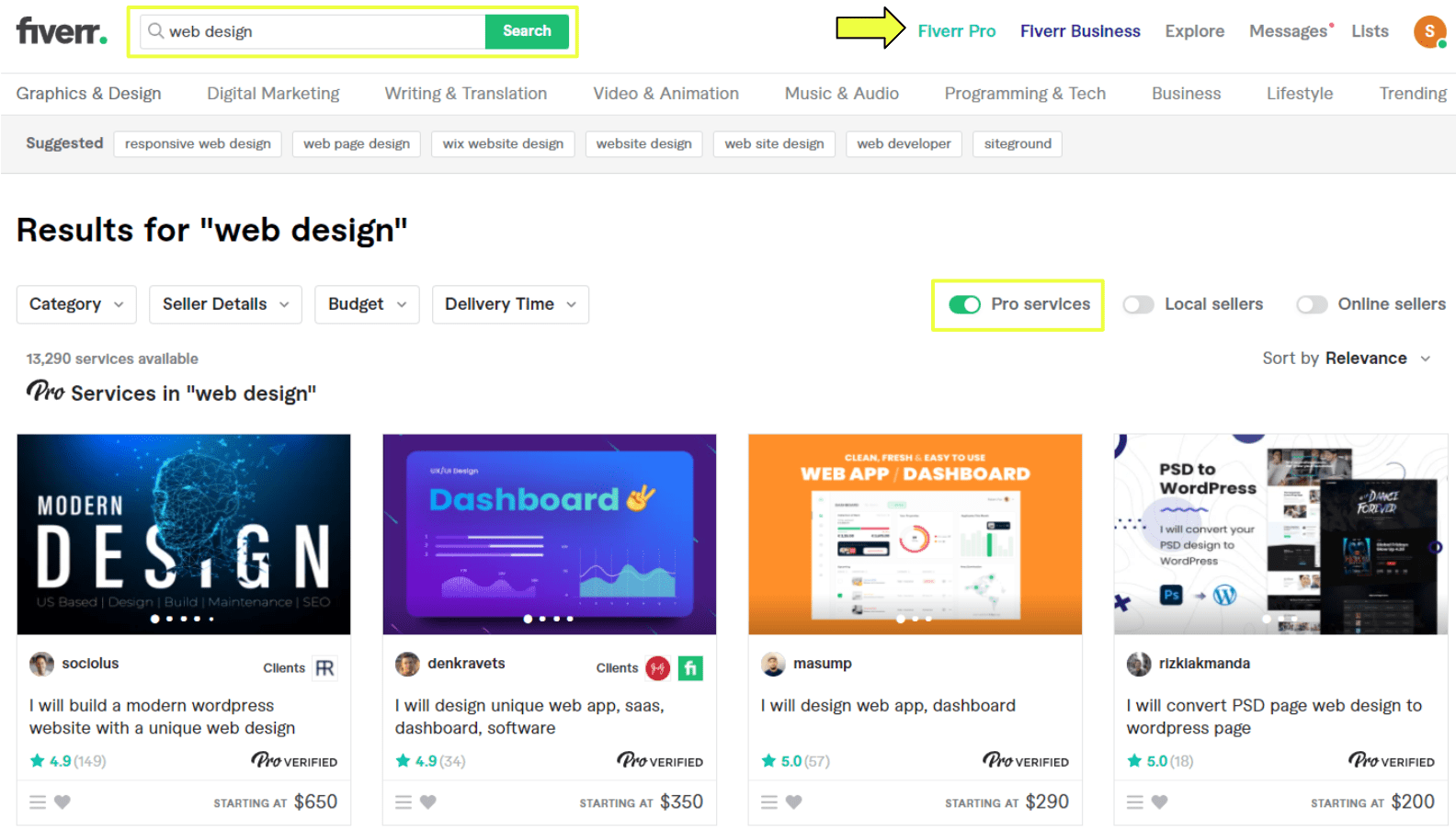In the image, we observe a detailed snapshot of a web page belonging to Fiverr, a freelancing platform. The platform name "Fiverr" is displayed in lowercase, spelled F-I-V-E-R-R, in a black font with a green dot following it. The search bar, which is green, contains a yellow-highlighted search term "web design" alongside a magnifying glass icon.

Additionally, a graphic arrow directs attention to "Fiverr Pro," written in light green font. Nearby, "Fiverr Business" is featured in a blue font, and options like "Explore," "Messages," and "Lists" are displayed in gray font. An orange profile button with the letter 'S' indicates the user is online with a green dot.

At the top, several navigation tabs are visible, labeled as Graphic & Design, Digital Marketing, Writing & Translation, Video & Animation, Music & Audio, Programming & Tech, Business, Lifestyle, and Trending.

Finally, four different programs are showcased on the page:
1. "Modern Design" characterized by blue and black colors.
2. "Dashboard" featuring light blue and purple hues.
3. "Web App Dashboard" presented in orange and white.
4. "NPSD to WordPress" displayed in black and white.